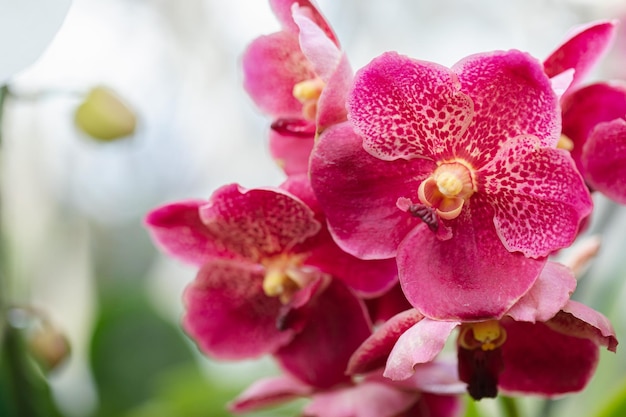In this vivid rectangular photo, the primary focus is on a cluster of seven large, vibrant flowers that closely resemble the color of red roses, but with hues leaning towards bright pink. Each flower boasts an intricate yellow center, characterized by a fascinating stamen structure that includes ring-like shapes topped with arched bows. Surrounding these magnificent blooms, some petals show a striking white discoloration reminiscent of leopard spots, adding further intrigue and uniqueness. The blurred background accentuates the sharp clarity of the main flowers, revealing a glimpse of green leaves and possibly more white flowers of the same variety on the left-hand side. This composition emphasizes the healthy and bright nature of these beautifully detailed and captivating flowers.